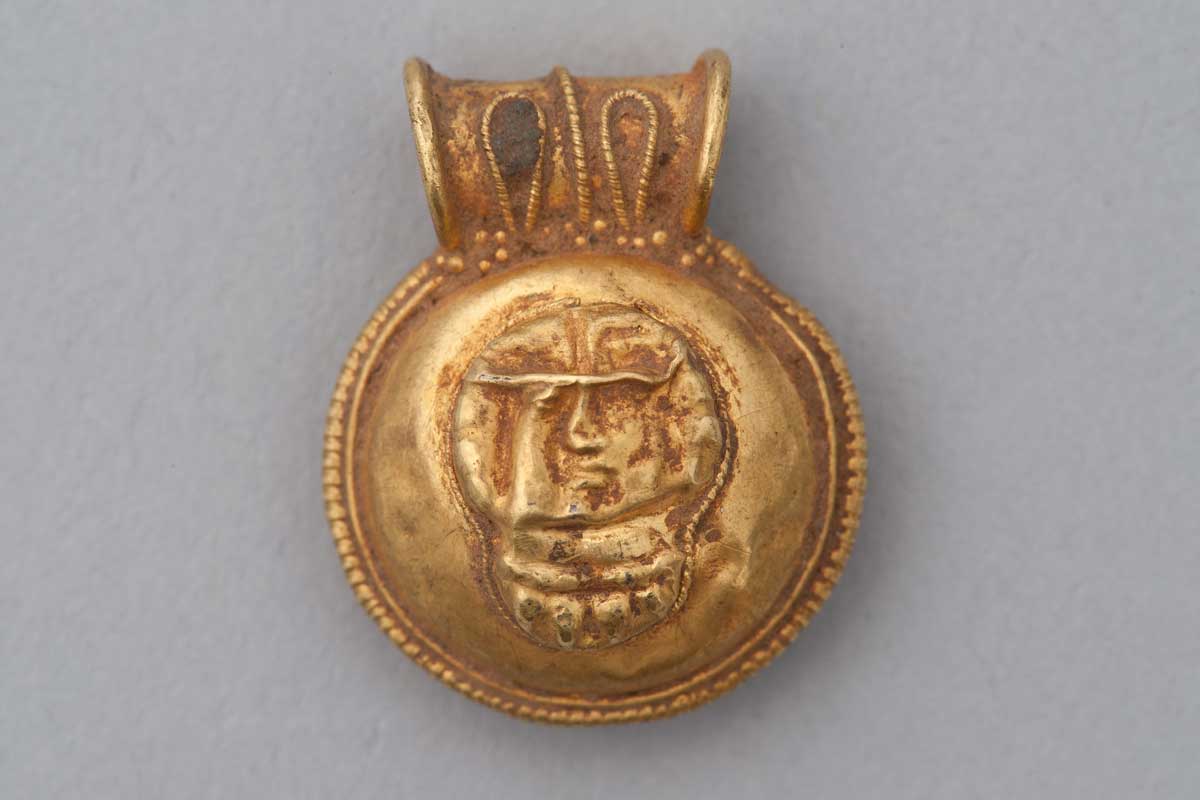The image depicts an intricately designed, circular gold charm set against a pale gray background. At the center of the charm, an engraved human face is prominently featured. This detailed face is surrounded by a border decorated with numerous tiny golden beads, creating a striking frame. The charm is topped with a ring-shaped or hook-like feature, likely designed to attach to a chain. This top section includes a central line flanked by two loop-shaped patterns, adding to the ornament's complexity. Despite its gold composition, the charm appears aged and weathered, exhibiting signs of rust and scratches. The lack of reference objects in the image makes it challenging to determine the charm's exact size.